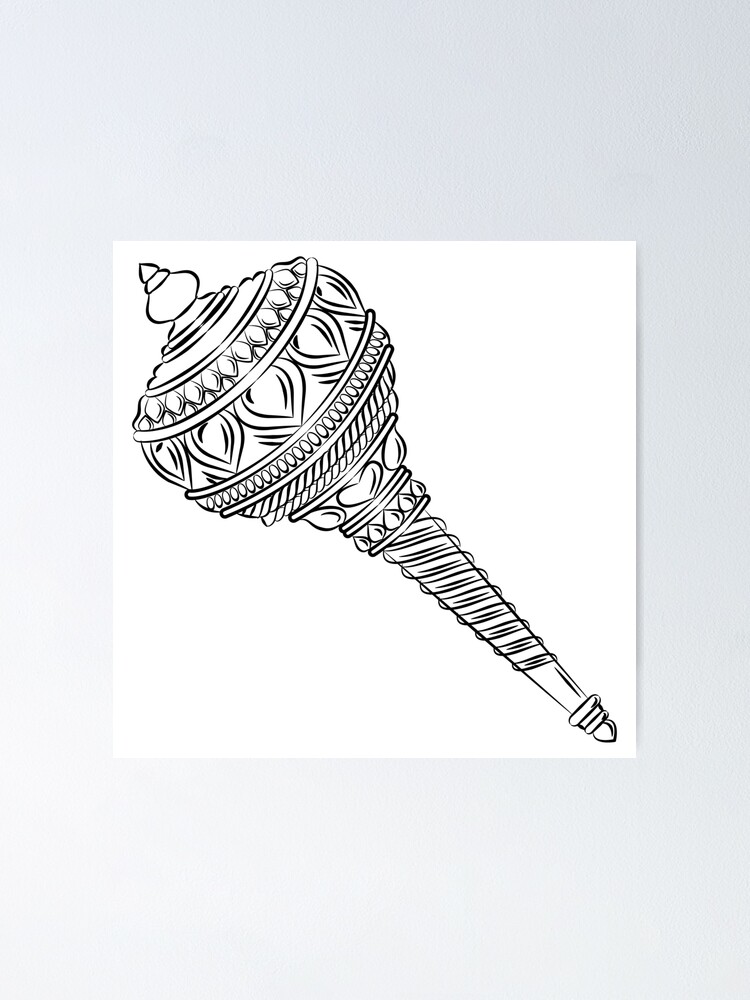The image is a detailed black and white line drawing or vector art of a scepter with a diagonally positioned figure on a plain, light gray background. The scepter features a handle resembling an ice cream cone, adorned with spiraling coils. The top of the scepter transitions into a complex spherical bulb, decorated with various patterns. Notably, the bulb has sections divided by horizontal lines, each containing different decorative elements: teardrops, hearts, twisted bands, and small ovals. Above the bulb, the structure tapers into a small, pointed tip that resembles a snowman's form, with progressively smaller sections culminating in a pointed top. The intricate design culminates in a finely detailed, ornamental scepter with a medallion-like shape at both the top and bottom ends.